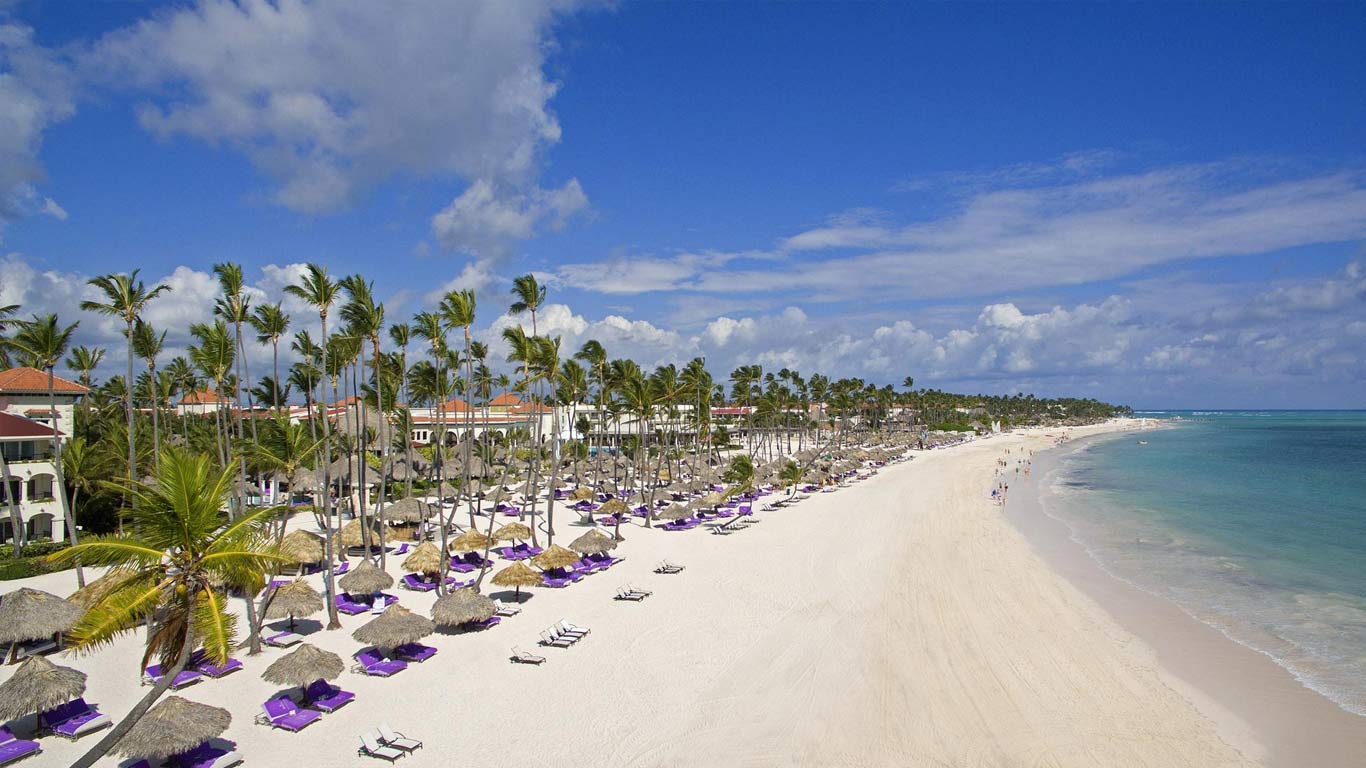The image is an aerial photograph of a beautiful, tropical beachfront. On the right side of the image, the calm, light blue ocean water gently laps against the very light tan sand of the beach, which curves to the right as it stretches into the distance. The sky above is a rich, dark blue, accented with some white, wispy clouds on the left side and a cluster of puffy white clouds on the horizon.

The left side of the image features rows of tiki, thatch umbrellas with purple loungers beneath them, stretching along the beach. Each umbrella shades a pair of padded purple beach beds, arranged in at least three visible rows and possibly extending up to twelve rows. Behind the umbrellas, numerous tall palm trees rise up, creating a tropical canopy. Further in the background, white buildings with terracotta shingled roofs are visible among the palm trees.

The beach is sparsely populated, with only a few small figures seen walking along the shoreline in the middle distance. The scene captures the serene and inviting atmosphere of this tropical paradise, with plenty of open space and a peaceful ambiance.